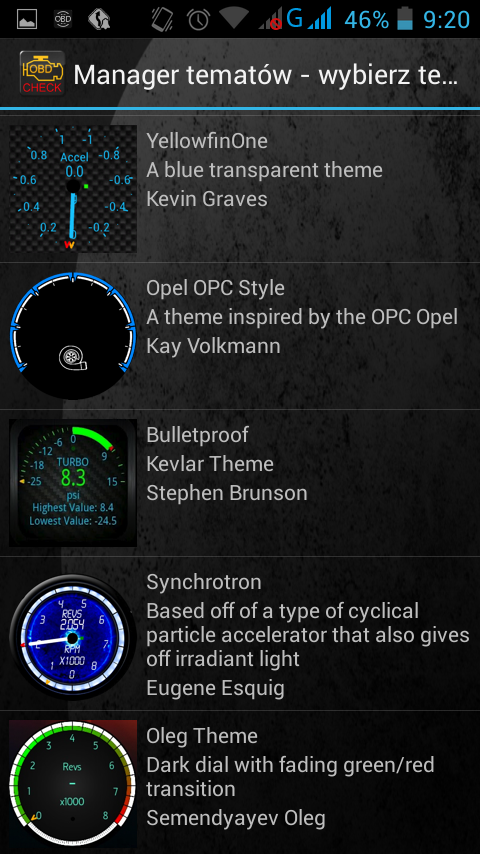The image is a detailed screenshot from a smartphone in dark mode, showing a grayish-black background. At the top, the screen displays the time as 9:20 PM and the battery level is at 46%. Several small icons indicating the phone's status—including battery percentage, signal strength, and the phone being set to vibrate mode—are visible at the top. Below these, there is a list of different themes for display dials, each with its own description. The themes include YellowFIN1, a blue transparent theme, Opal OPC style inspired by Kay Volkman, Bulletproof featuring a Kevlar theme by Steven Brunson, Synchrotron based on a cyclical particle accelerator by Eugene Esquig, and OLEG, a dark dial featuring a green to red transition. To the left of each description is a visual representation of the corresponding dial.